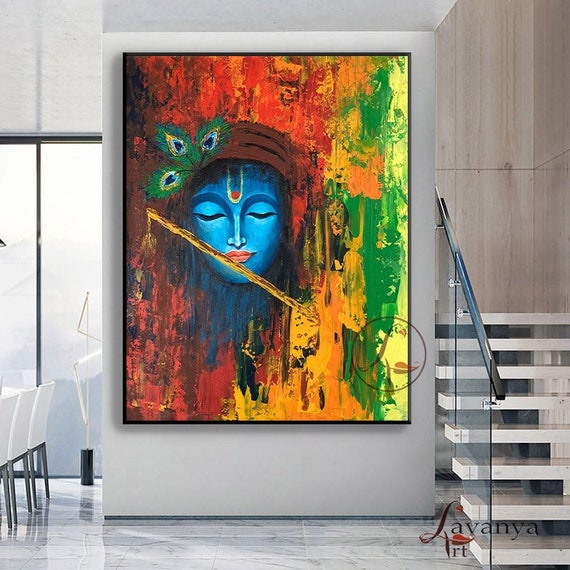The image depicts a bright, modern interior space, likely an art gallery or high-end apartment, highlighted by white and gray marble flooring with delicate gray streaks. Prominently featured is a striking painting of a woman with blue skin and red lipstick, set against a vibrant, abstract background that includes hues of red, orange, yellow, and green. The artwork incorporates peacock-like leaves emerging from her brown hat. Below the painting is a logo reading "Savannah Art." On the right side of the room, sleek white steps with a glass frame and metal railing appear to float, leading up to a second level with large glass windows. On the left, a partially visible table is accompanied by elegant white chairs. The overall atmosphere exudes modern elegance with its clean lines and sophisticated use of color and space.